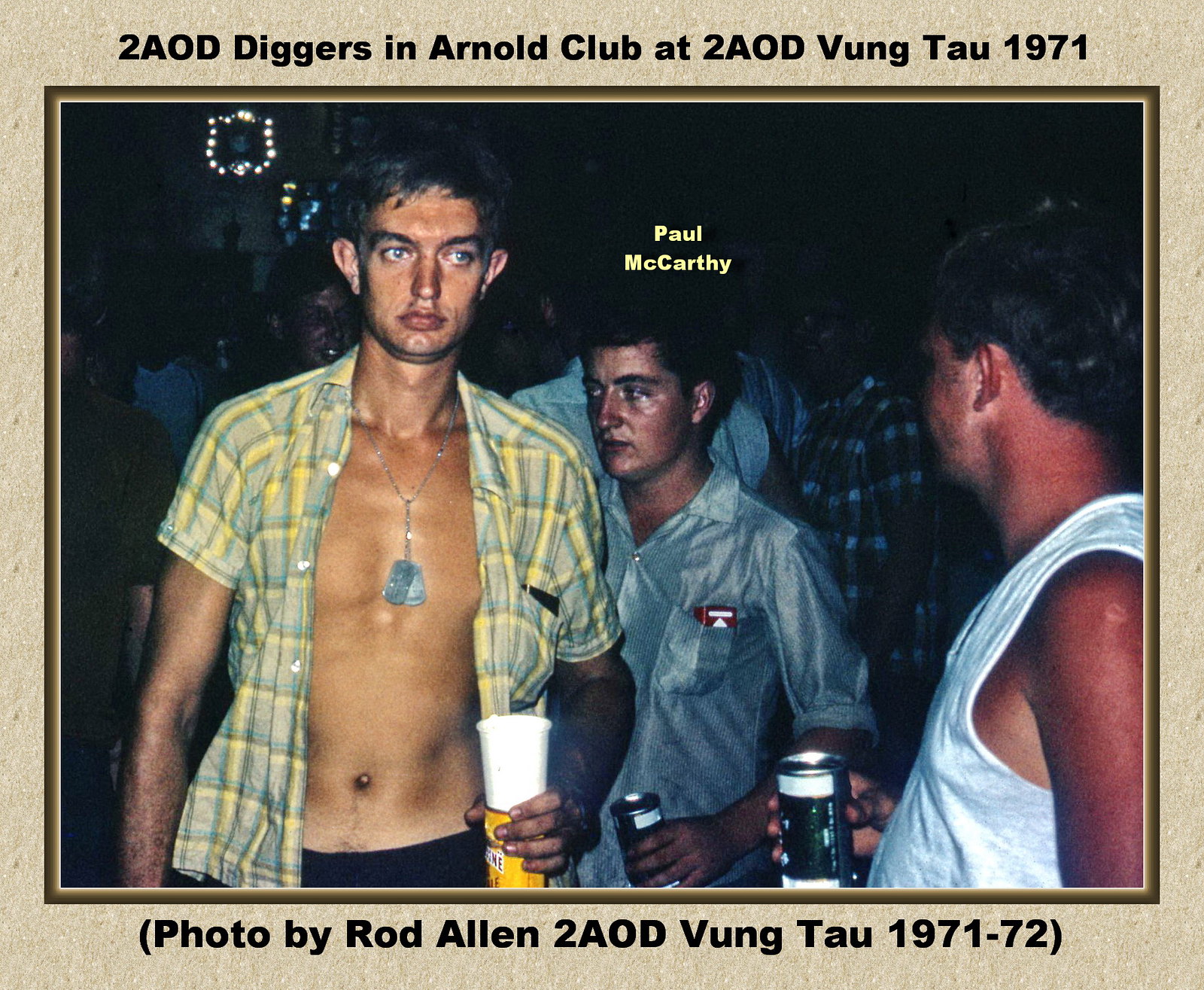This is a detailed photograph of three army soldiers relaxing in the Arnold Club at 2AOD Vung Tau in 1971, captured by Rod Allen. The top of the photo reads "2AOD diggers in Arnold Club at 2AOD Vung Tau 1971," and the bottom caption notes it is a "photo by Rod Allen 2AOD Vung Tau 1971-72." In the foreground, on the left, stands a tall, white male soldier dressed in a yellow plaid button-down shirt, open to reveal his chest, medals, and dog tags. He holds a drink in his left hand and sports black pants. Behind his left shoulder stands a smaller soldier with dark hair, wearing a silver-gray button-down shirt with a pack of cigarettes in the pocket. Above his head, in yellow letters, it reads "Paul McCarthy." The third soldier, positioned to the right, is also a white male with dark hair, wearing a white sleeveless shirt and holding a beer can in his right hand. The background shows more men enjoying the club atmosphere. The photograph has a tan border, accentuating the era and setting of the image.